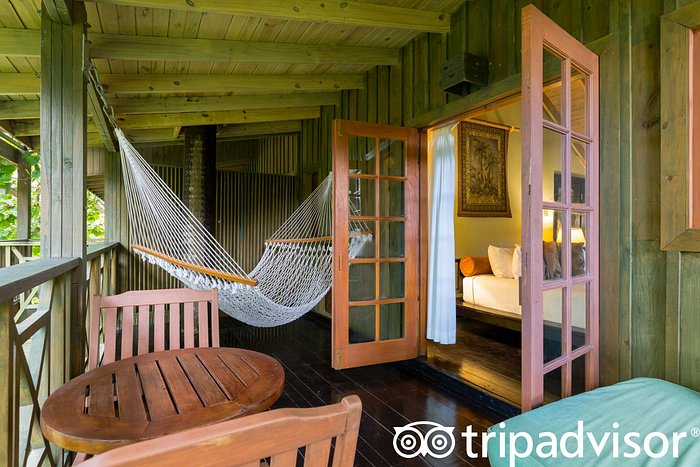This image, likely a promotional photograph for a rental property listed on TripAdvisor, showcases a beautifully designed porch area of a cabin or small home. The covered patio features well-crafted, stained wood in a mix of greenish tones, with a dark floor and lighter wooden beams, creating a harmonious blend of natural colors. On the left side of the porch, there is a small table accompanied by two wooden chairs, perfect for outdoor dining or relaxation. Towards the back, a white net hammock is suspended, inviting guests to unwind in comfort.

On the right side of the image, padded seating provides another comfortable spot for relaxation. Double French doors, adorned with glass panes and white curtains, open up to the cozy bedroom inside. This room is tastefully decorated with pillows, including a noticeable orange pillow, white sheets on the bed, and a painting or wall hanging above the headboard. The wooden doors leading from the bedroom to the patio have a pinkish hue, adding a charming touch to the overall aesthetic. The combination of natural wood and subtle painted accents contributes to the space's inviting and serene atmosphere.